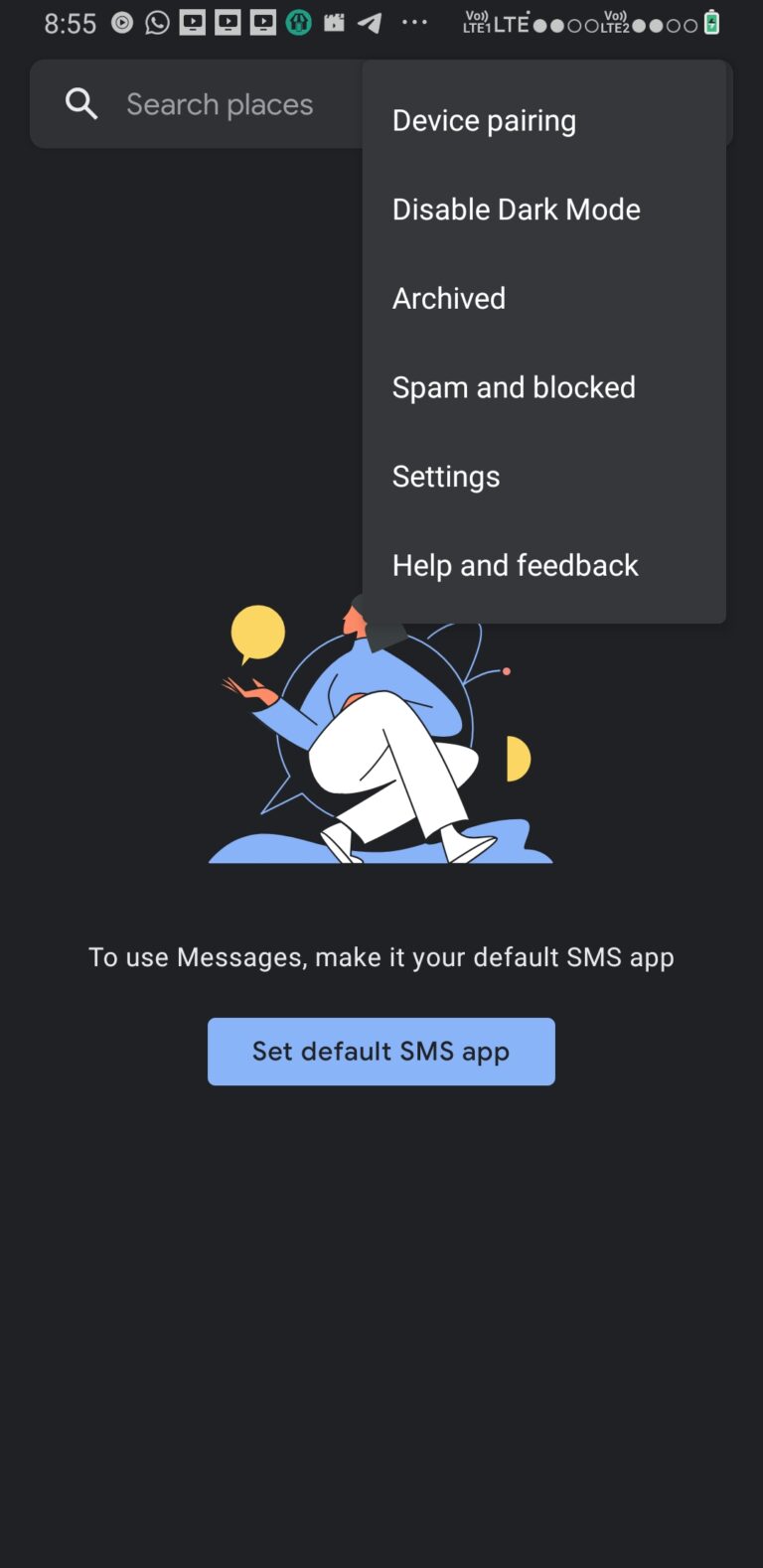The image shows a cellphone screenshot with the text message app open in dark mode. Overlaid on the upper left side of the screen is a settings panel displaying multiple options: 'Device pairing,' 'Disabled dark mode,' 'Archived,' 'Spam and blocked,' 'Settings,' and 'Help and feedback.' The reason the settings panel is open appears to be for the activation or usage of dark mode. The phone screen includes a status bar displaying several icons, indicating active downloads, open apps, active phone, and location services, suggesting this is a newly set up device.

The main view of the text message app shows an empty message box with a prompt stating, "To use Messages, make it your default SMS app." Below that prompt is a blue button labeled "Set default SMS app." At the top of the screen, a search bar displays the placeholder text "Search places." This detailed setup process indicates that the user is configuring their phone, likely a new one, for the first time.